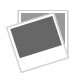The image depicts a rectangular, full-color photograph featuring a predominantly red and peach-colored abstract object with accents of brown, black, and white. The object starts from the lower right-hand corner and extends towards the center of the frame, set against a blurry gray and white background. The object has a distinctive, hollowed-out area that seems to be black or brown on the inside. It features a shape reminiscent of a neck and shoulders, with a small white squiggly line around what would be considered the neck area. The bright, lacquer-like exterior includes both red and peach tones, and there appears to be some damage on the left-hand side.